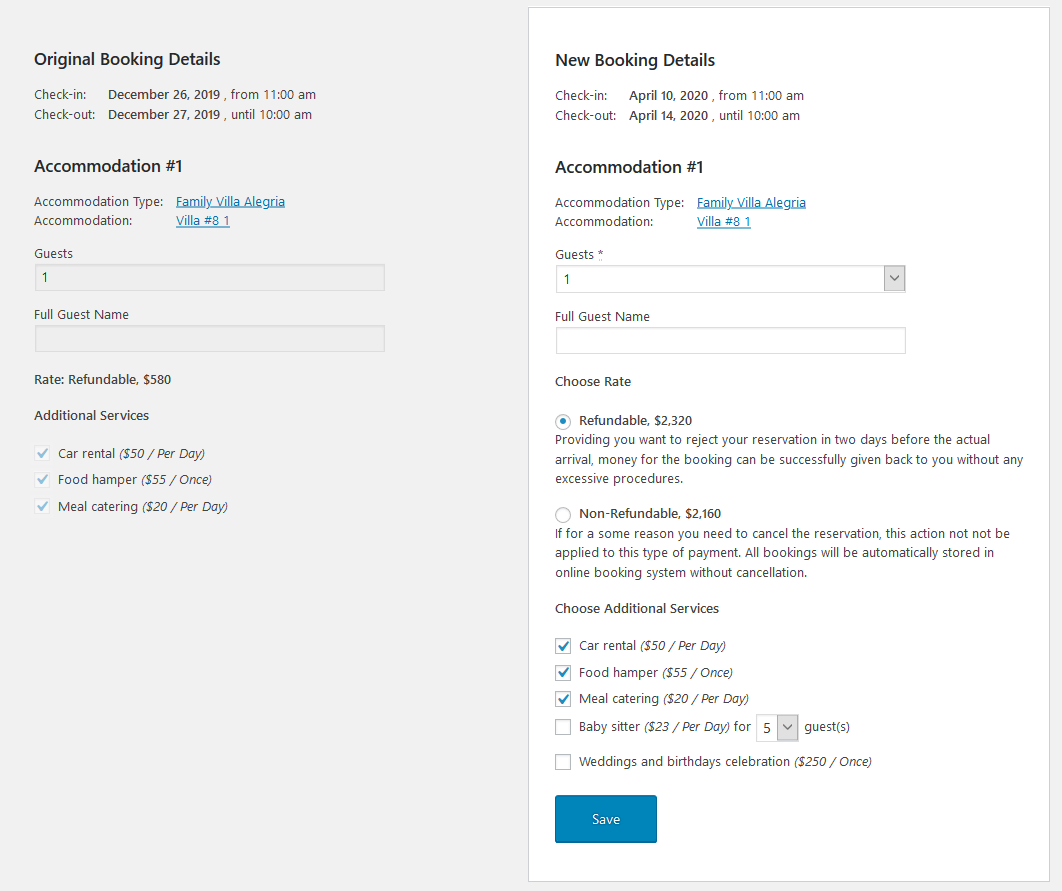This image showcases a booking page detailing original and revised booking information for a trip. Initially scheduled for check-in on December 26, 2019, the reservation included accommodation for one guest at a refundable rate of $580. Additional services such as car rental, food hamper, and meal catering were also listed, though displayed in a light gray font, making them less prominent against the small black text.

On the right-hand side, the new booking details are highlighted in white font. The revised booking now accommodates a stay from April 10 to April 14 at the Family Villa Alaguerra for one person. This updated reservation is refundable at a rate of $2,320, provided the cancellation is made within two days. The revised booking maintains the need for car rental and meal catering services. Overall, the form is neatly organized, presenting all essential information in a streamlined manner.